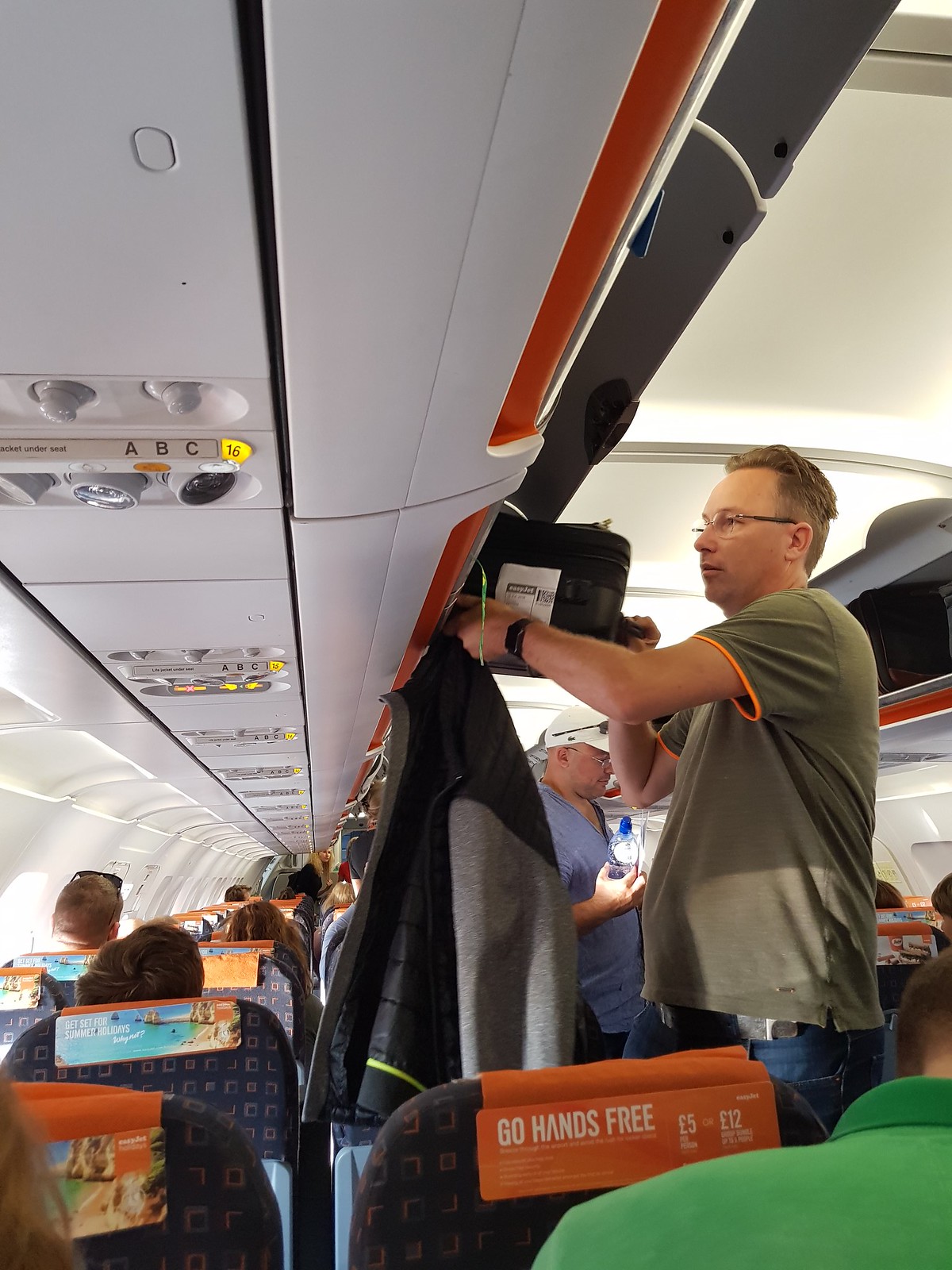In this detailed photograph taken inside a passenger airplane, a young man with light brown hair, wearing glasses, a green t-shirt, and blue jeans, is seen carefully rearranging his belongings in the overhead compartment. He has a dark letterman's jacket with grey sleeves draped over his left hand and a black wristwatch or smartwatch on his wrist. He appears to be focused on handling his dark-colored carry-on suitcase with his right hand. The interior of the plane is clearly visible, with rows of seats extending into the background where numerous passengers are still seated, visible by the backs of their heads. There is a small in-flight advertisement on the headrests that reads "Go Hands Free," accompanied by a serene beach scene. The overhead lights and controls are also visible, adding to the typical airplane ambiance. On the lower right, an indistinct man can be seen in a green shirt, partially out of frame.